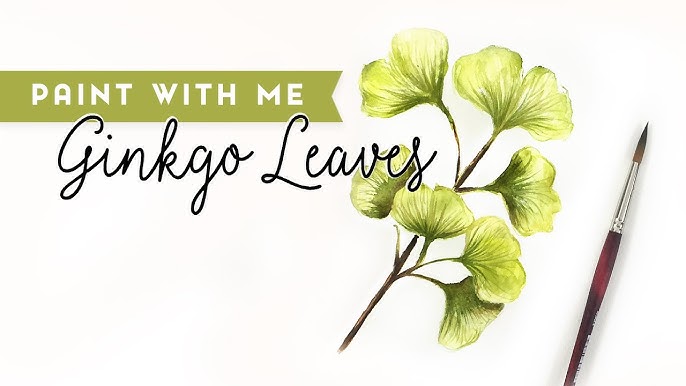This detailed painting, possibly an advertisement, features a prominent green flag in the upper left corner with white text stating "Paint with Me." Directly beneath this, in elegant black cursive, reads "Ginkgo Leaves." The focal point of the artwork is a diagonal arrangement of seven ginkgo leaves, depicted in very light green hues, stretching from the lower left to the upper right behind the text. These ginkgo leaves are attached to a brown stem and exhibit subtle white tips. Complementing this botanical element is a painted image of a paintbrush to the right of the leaves. The paintbrush boasts a red and brown handle capped with a silver ferrule, while its bristles show a gradient of tan to black. The entire composition is set against a crisp white background.